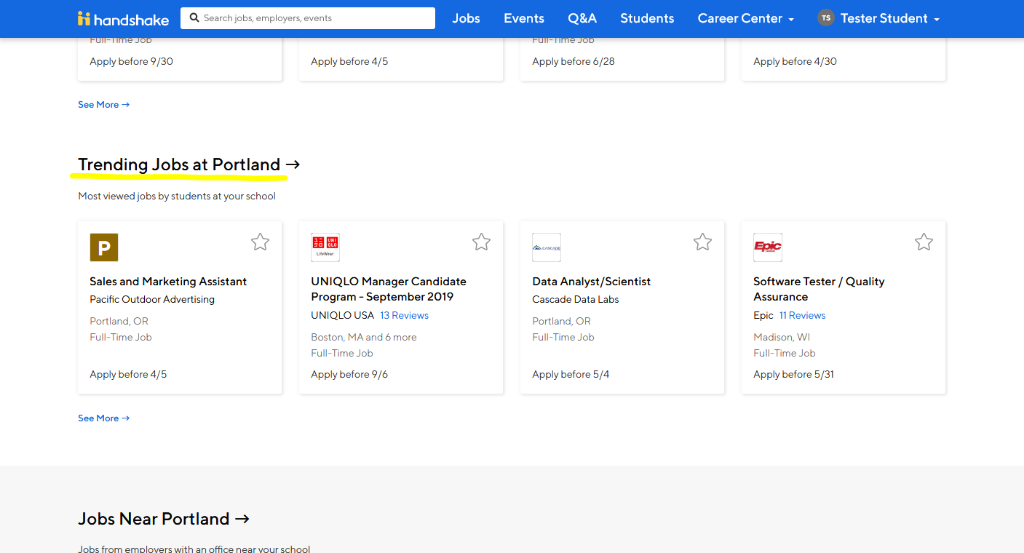**Caption:**

The image displays a webpage from the Handshake website featuring its distinct logo, which depicts two people shaking hands, situated on the left side. To the right of the logo is a search box and several tabs including "Jobs," "Events," "Q&A," "Students," and "Career Center," each with a drop-down arrow, as well as a "Tested Student" tab with a drop-down arrow.

Below these tabs are four truncated boxes with application deadlines. The deadlines read: "Apply Before 9/30," "Apply Before 4/5," "Apply Before 6/28," and "Apply Before 4/30." A "See More" option and a right-facing arrow follow the boxes.

Beneath this section is a highlighted and underlined heading in yellow, "Trending Jobs at Portland," followed by the text, "Most Viewed Jobs by Students at Your School." This section showcases four job listings, each in individual boxes:

1. "Sales and Marketing Assistant" at Pacific Outdoor Advertising in Portland, Oregon; a full-time position with an application deadline of 4/5. This listing includes a star icon indicating it can be saved.

2. "Manager Candidate Program, September 2019" at UNIQLO USA in Boston, Massachusetts, featuring 13 reviews and six more full-time job listings. The application deadline is 9/6. This listing also includes a star icon.

3. "Data Analysis/Scientists" at Cascade Data Labs in Portland, Oregon; a full-time position with an application deadline of 5/4. This listing includes a star icon.

4. "Software Tester/Quality Assurance" at Epic in Madison, Wisconsin, featuring 11 reviews. This is a full-time job with an application deadline of 5/31. This listing includes a star icon.

The section below these job listings is titled "Jobs Near Portland" with a right-facing arrow and the subtitle, "Jobs from Employer with an Office Near Your School."